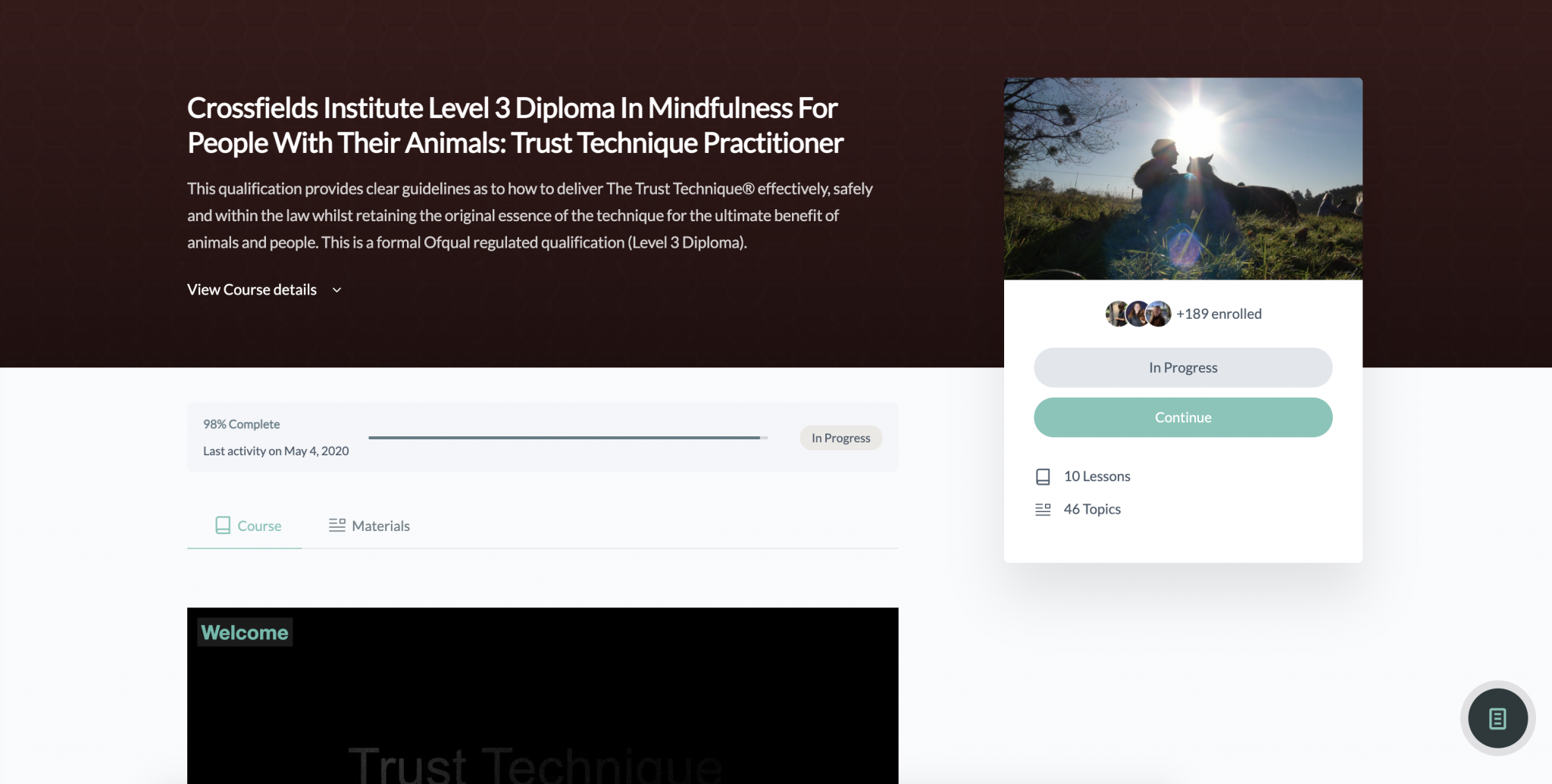The image showcases a website featuring detailed information about the "Crossfields Institute Level 3 Diploma in Mindfulness for People with their Animals: Trust Technique Practitioner." The top section of the website is styled with a dark brown background and white text. The prominent title reads, "Crossfields Institute Level 3 Diploma in Mindfulness for People with their Animals: Trust Technique Practitioner." It is followed by a descriptive paragraph explaining that the qualification offers clear guidelines to deliver the Trust Technique effectively, safely, and lawfully, while preserving the method's original essence for the benefit of both animals and people. The paragraph notes that this is a formally recognized Ofqual-regulated Level 3 Diploma. Below this description, there is an option to view course details.

Adjacent to the descriptive text, a box features an image of a person and an animal outdoors, with the sun shining behind them, though their details are not clearly visible. Within the same box on a white background, icons represent the people who have enrolled in the course, indicating "+189 enrolled."

Below the enrollment icons, there are two rounded buttons. The one on top is gray with the dark gray text "In Progress," and the button beneath it is a minty teal color with white text stating, "Continue." At the bottom of this box, the text informs users that there are 10 lessons and 46 topics included in the course.

In the main content area of the page, users can see the percentage of the course and materials that have been completed so far, providing a clear overview of their progress. The bottom half of the webpage transitions to a white background with mint and gray text, maintaining a clean and organized appearance.